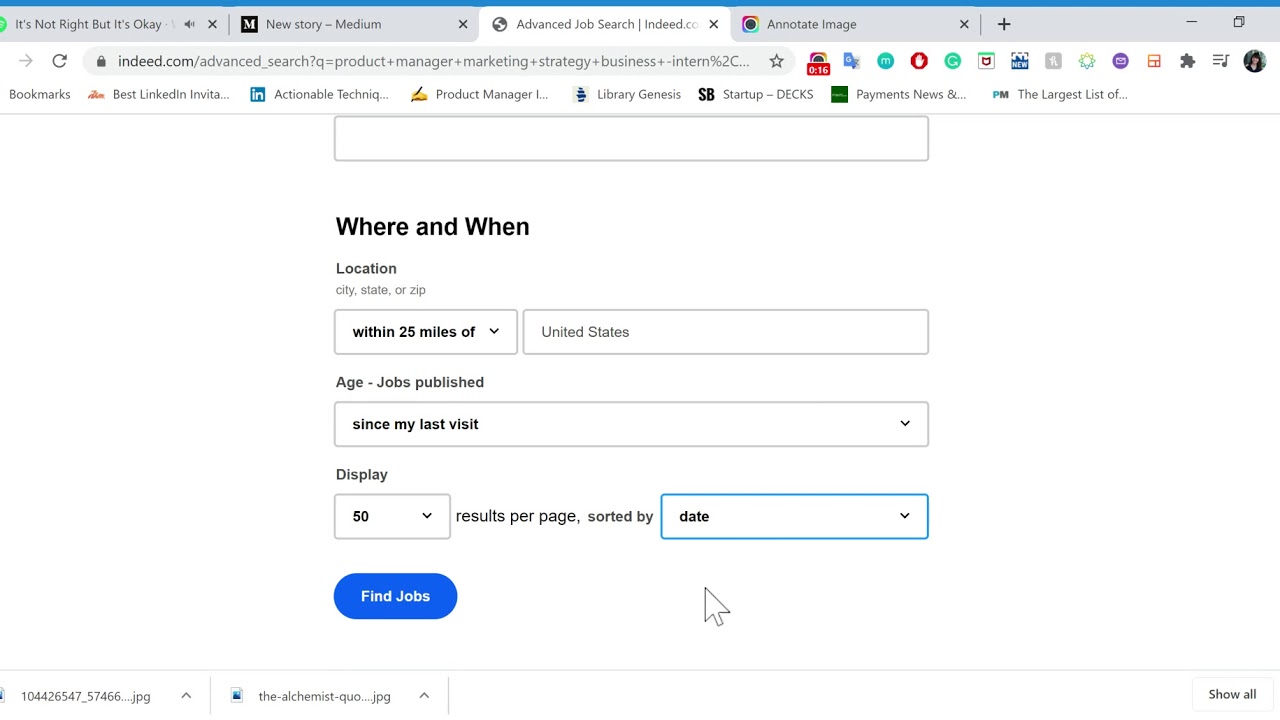The image depicts a Chrome browser with four tabs open. The tabs are titled: 
1. "It's Not Right but It's Okay" 
2. "New Story Medium" 
3. "Event Job Search - Indeed.com"
4. "Annotate Image".

The bookmarks bar displays several bookmarks labeled: 
1. "Best LinkedIn Actionable Techniques" 
2. "Product Manager"
3. "Library Genesis"
4. "Startup Decks"
5. "Payment News"
6. "The Largest List of".

Below the bookmarks bar, there is an empty input box. Below the box, the text "Where and When" appears, followed by fields labeled "Location City, State or ZIP" and a drop-down box with the option "within 25 miles of". To the right, there's a box labeled "United States". Beneath this section, additional fields are labeled "Age Job Published" with another box underneath that says "Since my last visit".